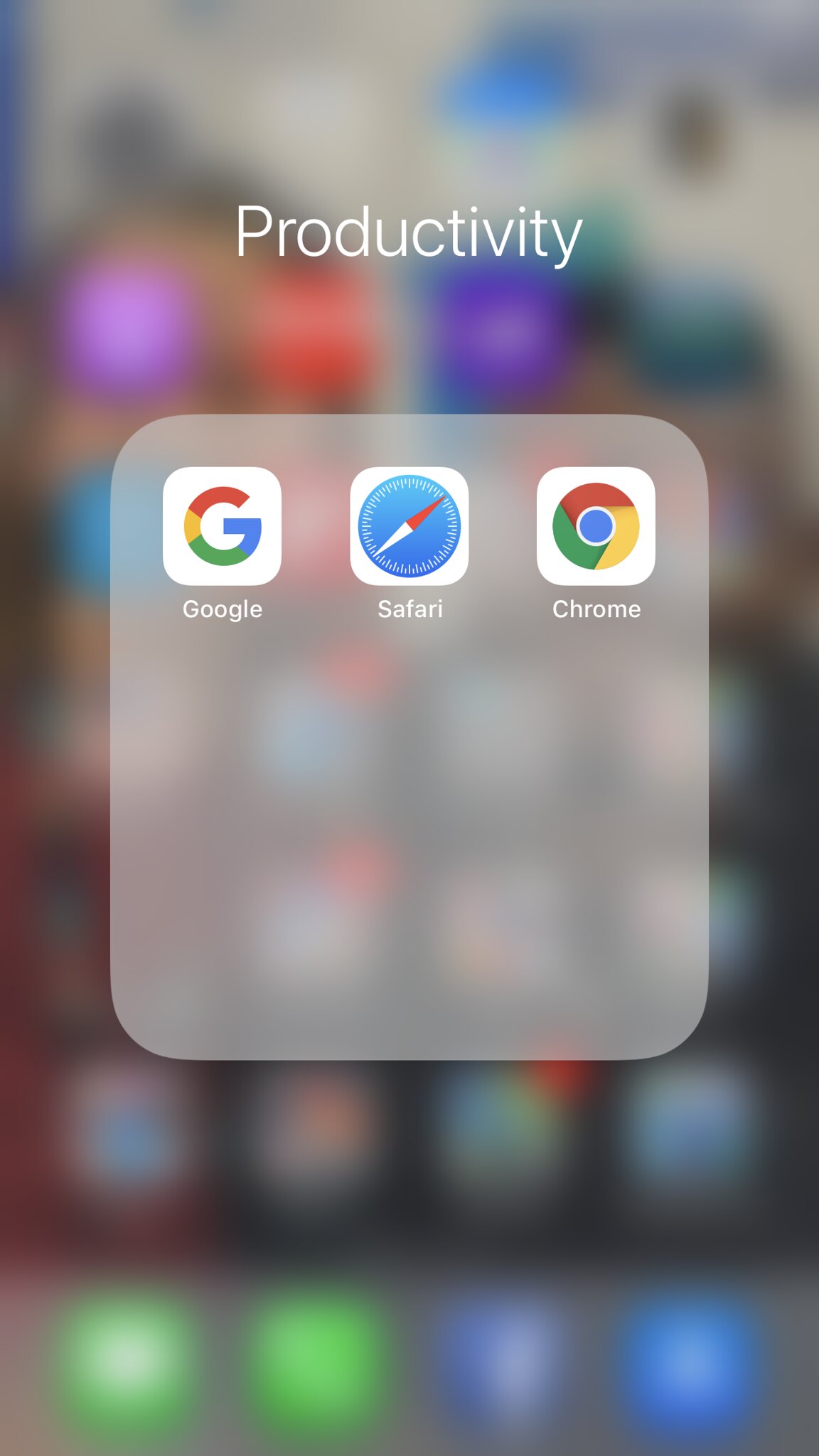This image is a screenshot from a smartphone, identifiable by its distinct rectangular shape and the visible app icons in the blurred background. Dominating the screenshot is a specific page labeled "Productivity," which is prominently displayed in white font at the top. Just below this heading, a sub-window is present, housing three essential app icons designed to enhance productivity.

The first icon on the left is the Google app, represented by a multicolored "G." Next to it, in the center, is the Safari icon, depicted as a blue dial with white scale divisions and a red and white compass-like pointer, signifying the Safari web browser. Completing the trio on the right is the Google Chrome icon, featuring its recognizable concentric circles with blue at the center, surrounded by green, yellow, and red segments.

The blurred background hints at the smartphone's main screen filled with other apps, although they remain indistinct due to the overlaying sub-window. This screenshot effectively highlights the "Productivity" section, showcasing the key apps Google, Safari, and Chrome in a clean and focused view.